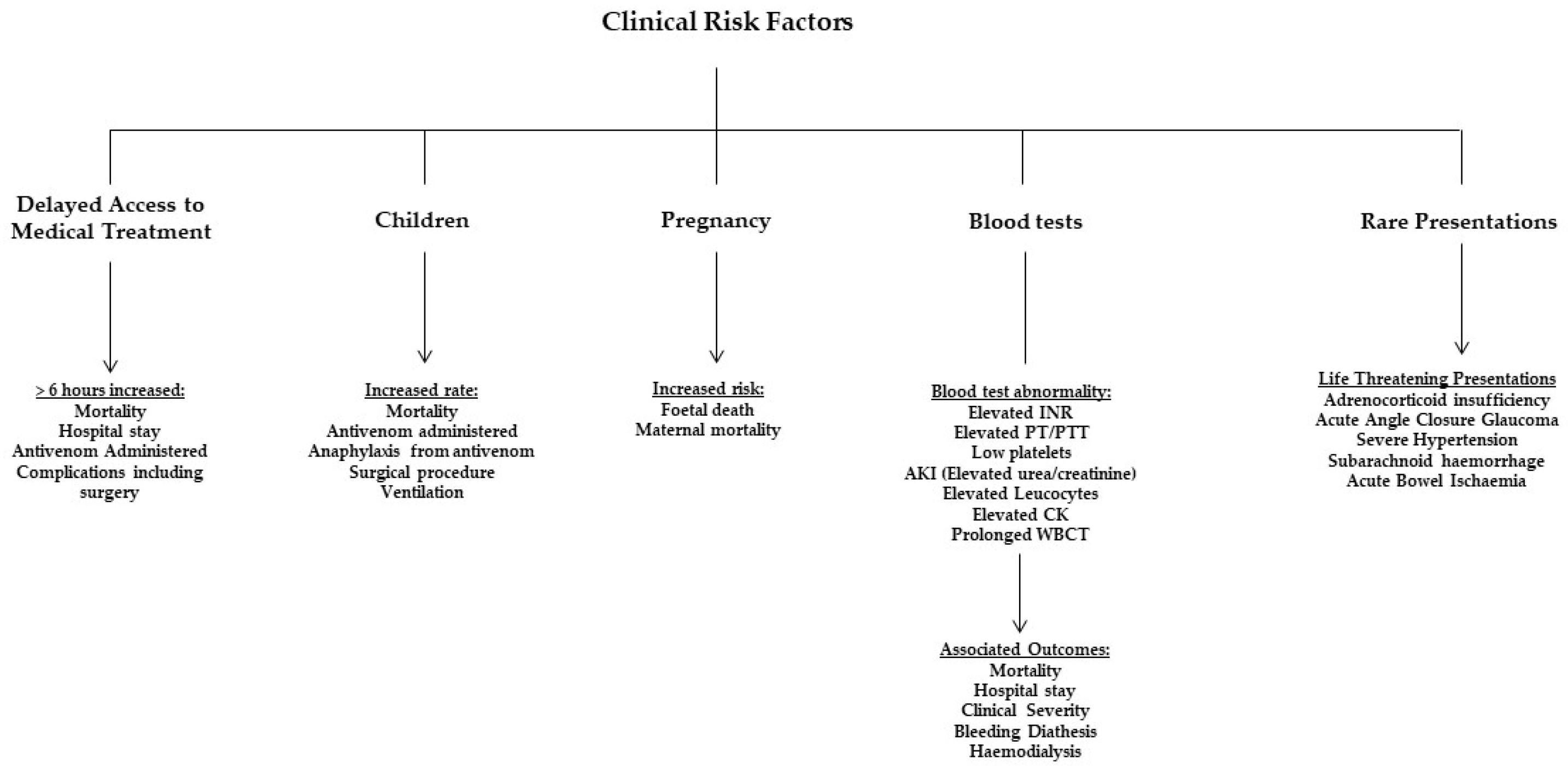This detailed flowchart, titled "Clinical Risk Factors," is presented on a white background with black text. Centrally positioned, the title "clinical risk factors" is prominent above the chart, which is rectangular and divided into five key categories, each with corresponding risk factors.

1. **Delayed Access to Medical Treatment:** Connected by an arrow, this section highlights risk factors such as increased mortality after six hours, extended hospital stay, the administration of antivenom, and the potential for complications requiring surgery.
   
2. **Children:** This section emphasizes the heightened risk of mortality, administration of antivenom, possible anaphylaxis from the antivenom, and the necessity for surgical procedures or ventilation.
   
3. **Pregnancy:** Here, the chart outlines the increased risks for both fetal death and maternal mortality.

4. **Blood Tests:** This category is further subdivided into various abnormalities, including elevated INR and PT/PTT, low platelets, AKI, elevated urea and creatinine, elevated leukocytes, elevated CK, and prolonged WBCT. The associated outcomes of these abnormalities are detailed as increased mortality, longer hospital stay, clinical severity, bleeding diathesis, and the need for hemodialysis.

5. **Rare Presentations:** This final section lists life-threatening conditions like adrenocortical insufficiency, acute angle-closure glaucoma, severe hypertension, subarachnoid hemorrhage, and acute limb ischemia.

Each category is meticulously linked by arrows, visually delineating the specific risk factors and outcomes related to each clinical scenario. This flowchart serves as a comprehensive guide to understanding diverse clinical risks in a medical context.